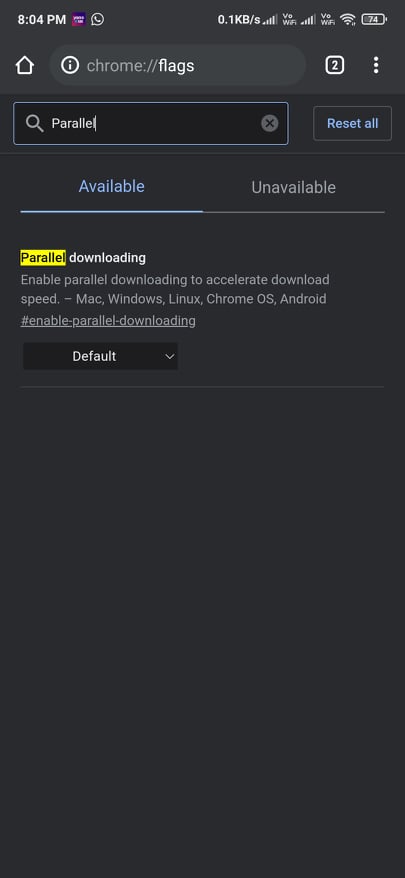This image is a screenshot taken on a cell phone at 8:04 PM. In the upper right corner, the WhatsApp icon and a battery indicator showing 74% are visible. The screenshot features the Chrome Flags page within the Google Chrome browser. At the top of the screen, there's a search bar that reads "chrome://flags." Just below the search bar, two icons are present: a box with the number "2" and an ellipsis indicating additional settings.

Directly underneath, there are two prominent options: one labeled "parallel," and next to it, a box labeled "Reset all." Below these options, two tabs are visible: "Available" and "Unavailable," with "Available" currently selected.

Further down, text reads "Parallel downloading," followed by a description: "Enable parallel downloading to accelerate download speed. Mac, Windows, Linux, Chrome OS, Android." Below this description, a link is labeled "#enable-parallel-downloading," with another mention of "Enable parallel downloading." Adjacent to the description, there's a dropdown menu labeled "Default."

This detailed screenshot captures a specific setting within the Chrome Flags page focused on the parallel downloading feature.